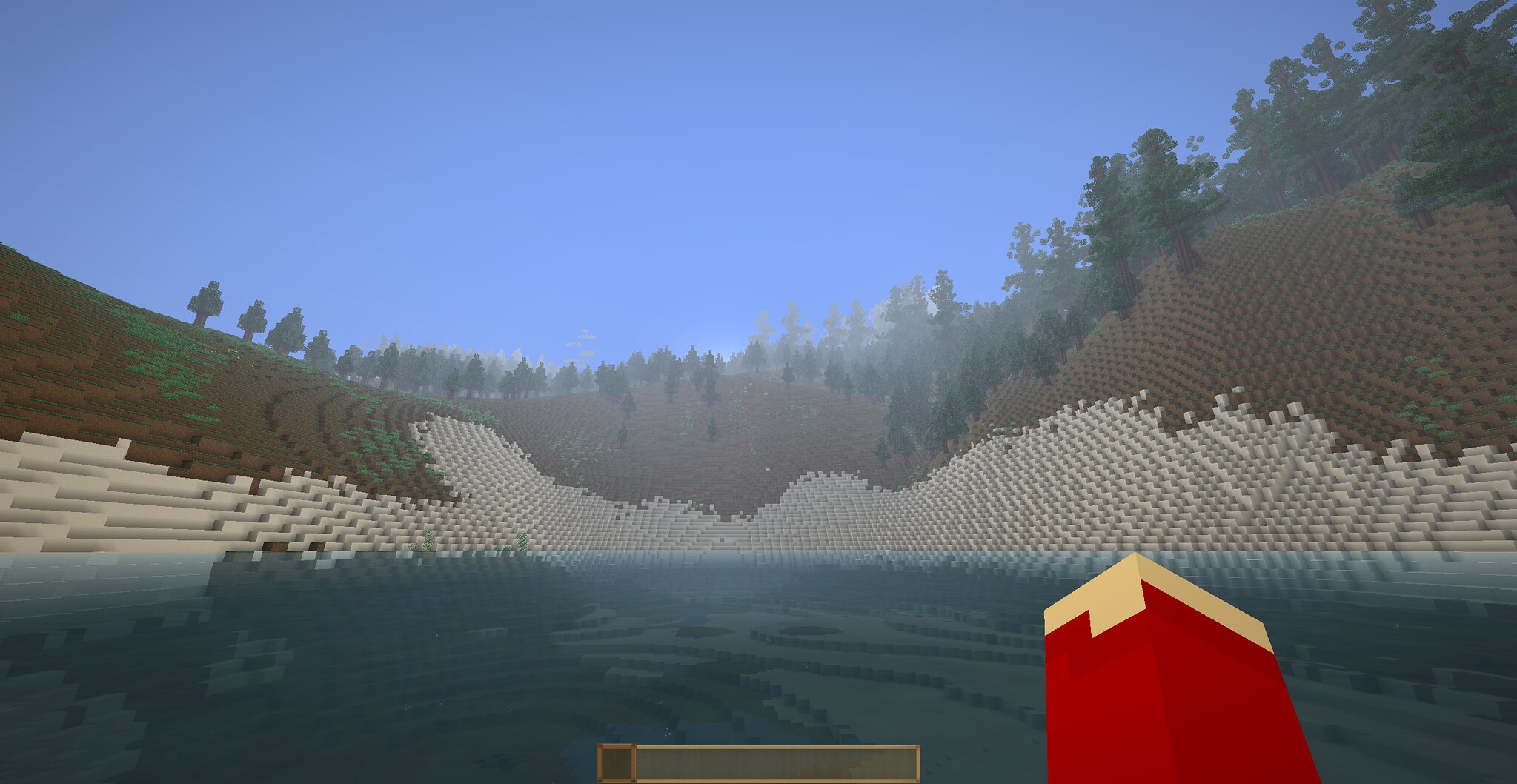The image depicts a detailed first-person perspective scene from Minecraft, enhanced with a texture pack that deviates from the standard, giving it a unique visual style. In the foreground, there is a body of water reminiscent of Lego blocks, characterized by a distinctive blocky appearance common in Minecraft terrain. On the right side of the frame, a red structure with a white tip, possibly resembling a chimney or a hand, juts out from the water. The coastline features a mix of white and gray blocks that simulate waves lapping against the shore. The landscape transitions sharply from sandy beaches to a steep, vertical incline composed of dark brown blocks, adorned with patches of green grass and dotted with pixelated trees, suggesting a lush, elevated valley. The scene is set against a clear blue sky, contributing to the vibrant and immersive environment.